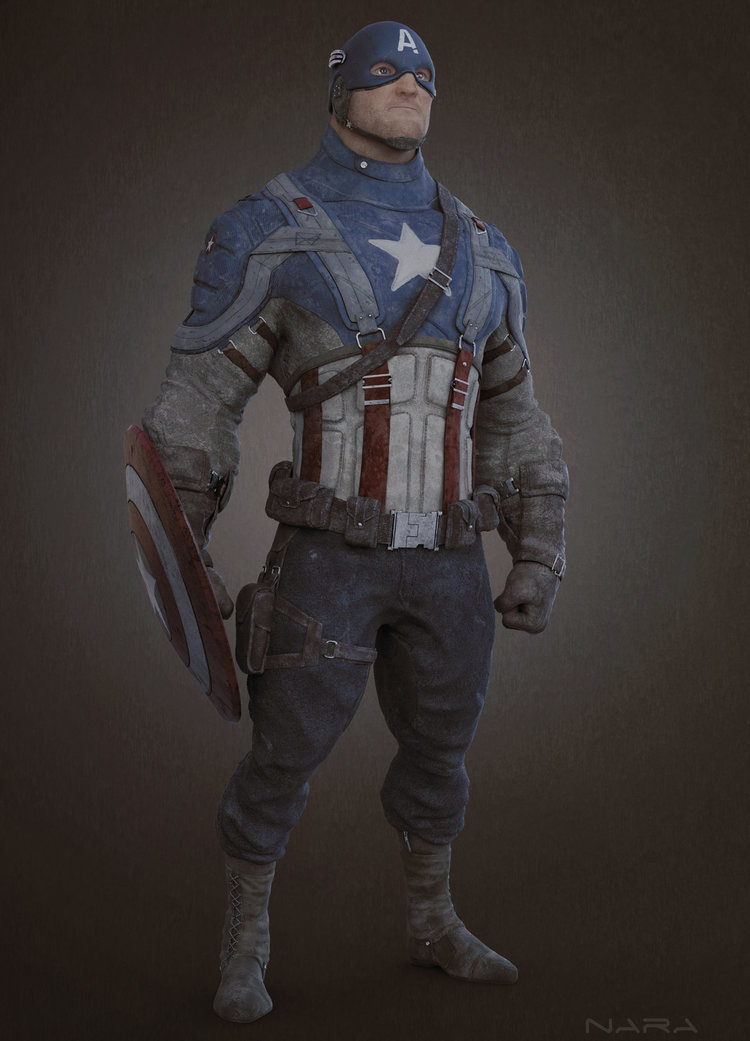This image depicts a vintage, highly detailed 3D statue of Marvel Comics' Captain America, distinctly showcasing elements from a bygone era rather than a modern interpretation. Captain America stands in a heroic pose, looking muscular and tough. He wears a blue helmet adorned with a prominent white capital "A" on his forehead. His mask reveals his lower face, including his nose, mouth, and chin, while covering his eyes and head.

His uniform features a striking combination of blue, gray, white, and red. The upper section of the uniform has a large white star centered on his blue chest with white and red stripes running down the middle of his abdomen. He has a utility belt around his waist and wears blue-black pants with black boots. Notably, he is equipped with a utility side pocket on his sleeves.

Captain America confidently holds his iconic shield in his right hand. The shield displays a design of concentric red and white circles, with a white star in the center. The image's detailed rendering and the superhero's striking pose suggest that it might be from a video game or a digital animation, created with high precision, possibly by an artist or studio named N.A.R.A (Nara).